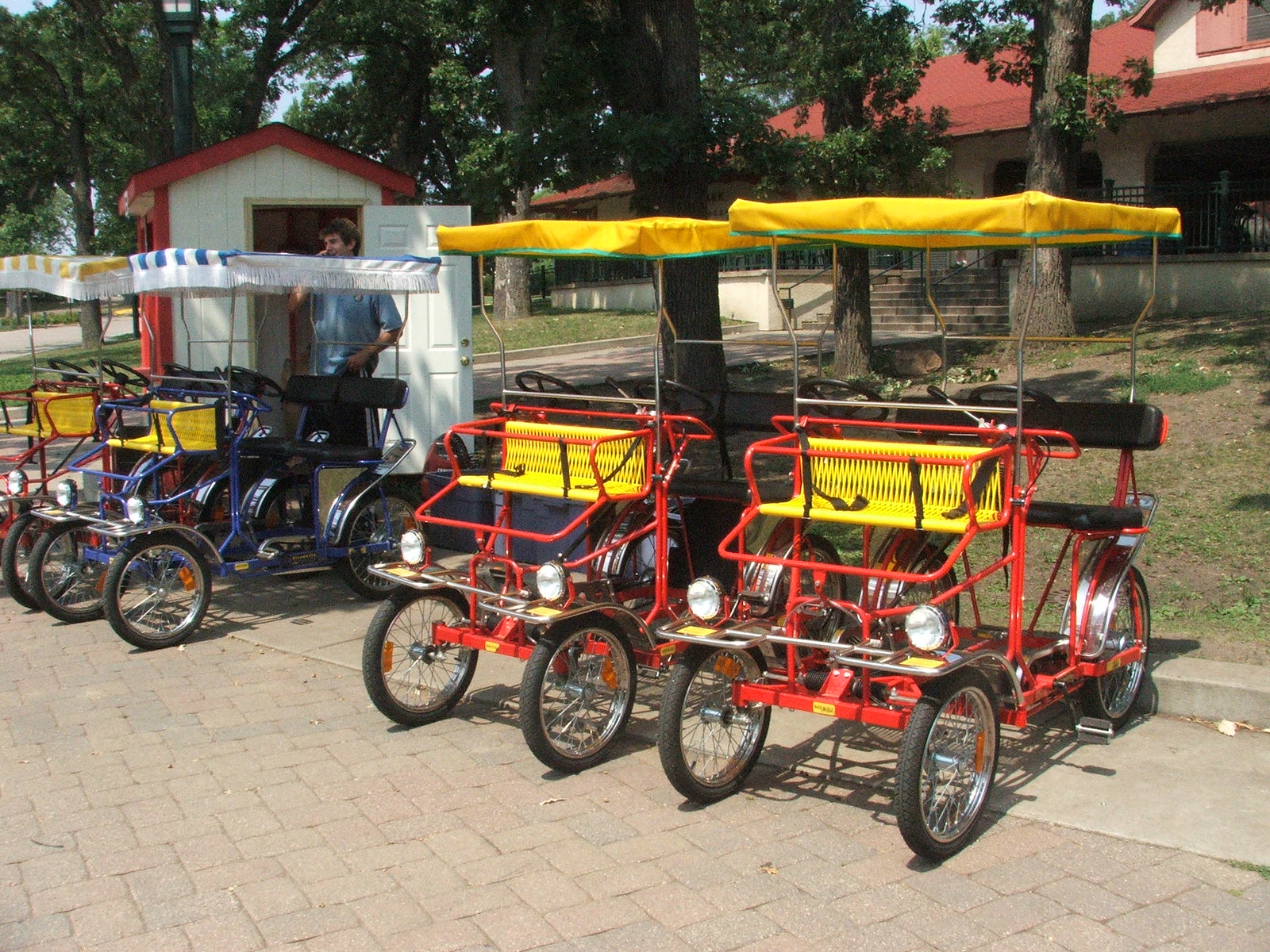In this vibrant outdoor setting, a digital photograph captures a single-story house with an attic, adorned with an orange and white facade and a red roof. The photo is taken on a sunny day, accentuating the lush green leaves of the numerous brown-trunked trees in the background. To the left of the house, there is a small white shed with a red roof, its door open, revealing a Caucasian man in a blue short-sleeved shirt and black shorts, holding a cell phone to his ear. He stands on a concrete walkway that includes steps leading up to the house. In the foreground, a gray brick road extends across the scene, hosting four unique two-person bicycles—each resembling a hybrid of a golf cart and a bicycle. The bicycles have vivid colors: two with blue frames and striped roofs (white and yellow, blue and white) positioned near the shed, and two with red frames and solid yellow roofs situated closer to the right side of the picture. The entire scene is bathed in bright sunlight, adding warmth to this picturesque, square-shaped image.